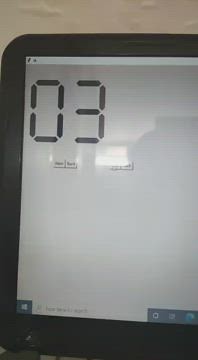This image captures a narrow, vertically rectangular frame with a composition divided between a light brown background in the upper section and the left side of a black-framed monitor filling the rest. The monitor's screen displays a white to off-white hue, reflecting a nearby window behind the camera. At the upper left corner of the screen, two digital numbers read '03', formed by black bar segments. Directly beneath the numbers, there are two small, indistinct selection buttons.